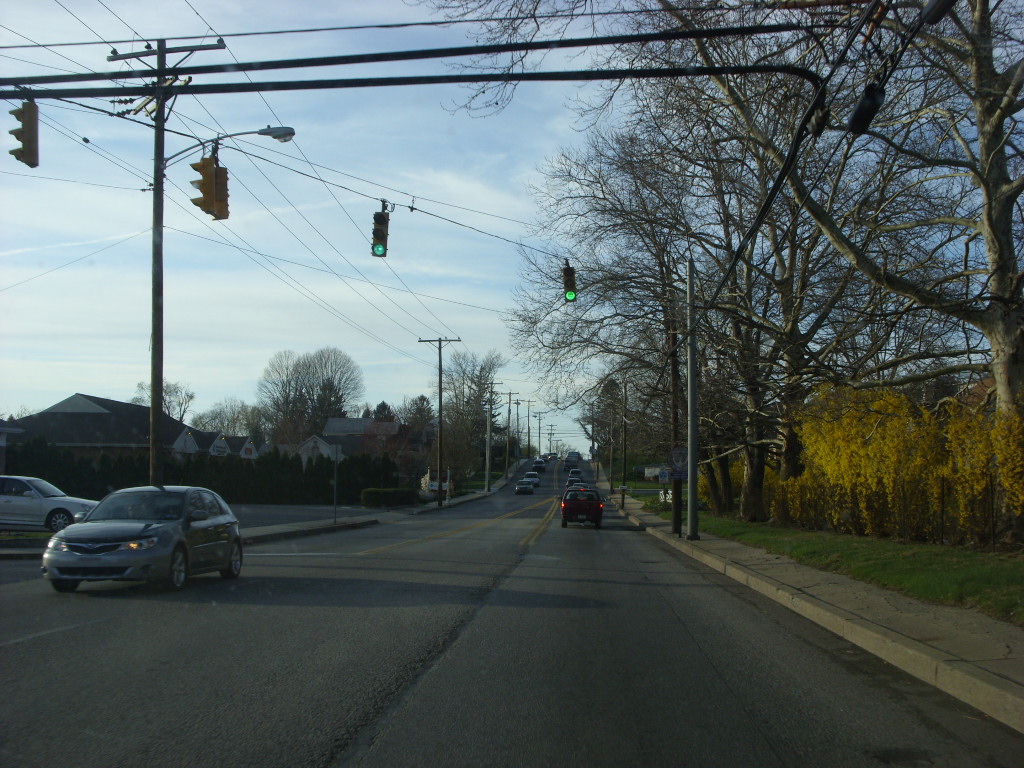The photograph captures a view from within the right lane of a two-lane street, looking straight down the road. The street features darker pavement. To the right, there's a sidewalk bordered by grass and smaller bush trees with yellow foliage, leading up to larger trees without foliage. Above the street, a line of four traffic lights, mounted on wires stretched across the roadway, displays green lights—two facing left and two facing towards the viewer. In the distance, ahead on the street, there’s the back of a car with visible taillights, while a gray car with its headlights on drives towards the photographer. Several other cars are also making their way towards the viewer, forming a line. On the left side of the image, adjacent to the roadway, there are rows of houses and possibly a strip mall further in the background, amidst several leafless trees. The sky above is a clear blue, dotted with wispy clouds, adding a serene backdrop to the urban scene. The image seems to be taken from either a vehicle or motorcycle, emphasizing the motion and perspective typically associated with travel.